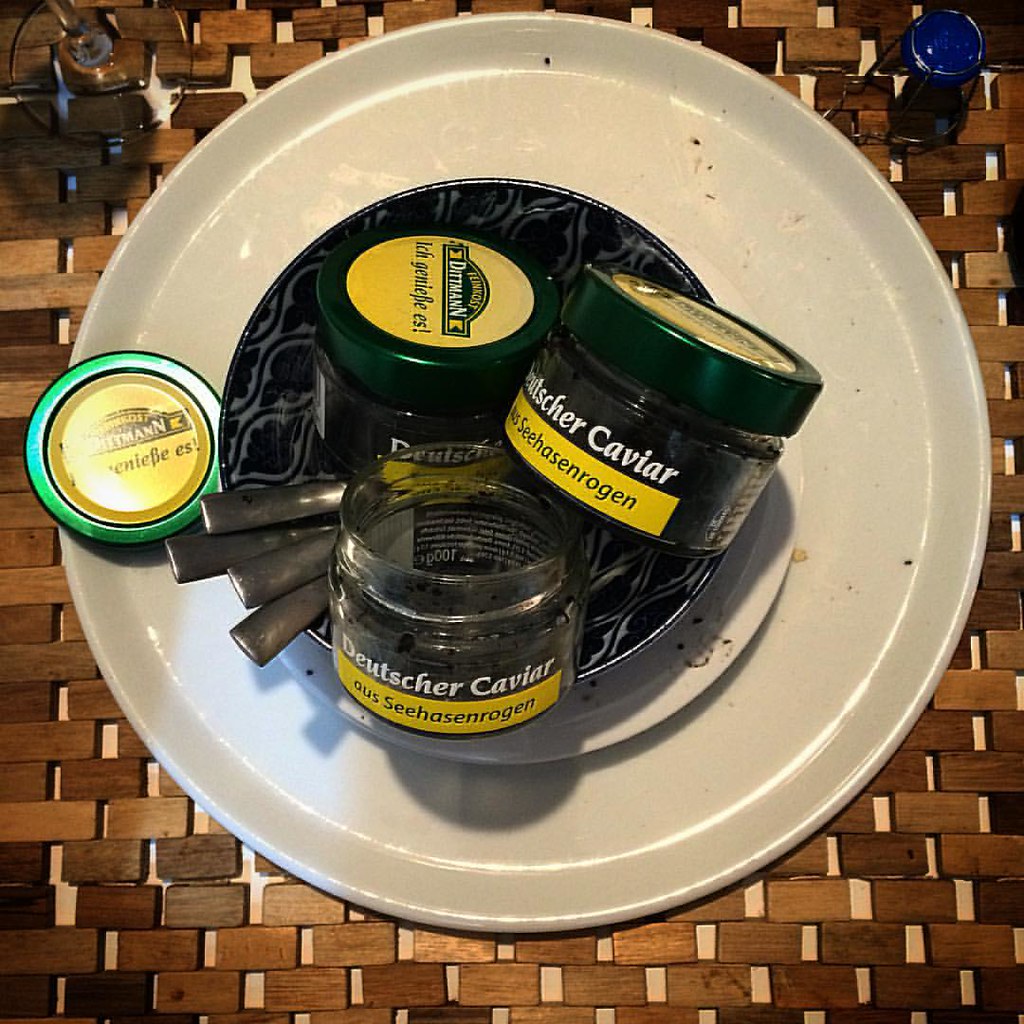The image depicts a detailed scene centered around an arrangement featuring caviar containers. At the forefront, a white plate laden with small black and brown smudges supports a second, smaller white plate marked with black traces of caviar. Atop this smaller plate rests an intricate black bowl adorned with diamond-shaped patterns, housing several utensils, likely four in total, though it's unclear whether they are spoons or forks. This bowl contains three caviar containers, labeled "Deutscher Caviar," with two containers featuring green lids and the third opened to reveal the black caviar inside. The open container’s lid resides on the white tray, which also exhibits similar black markings. This entire assembly is set on a rustic bamboo placemat composed of small interconnected wooden pieces. Visible in the background is some sort of electronic equipment, with a black power cord extending from one side. Additionally, a glass drinking cup is positioned to the left, completing the meticulously set scene.